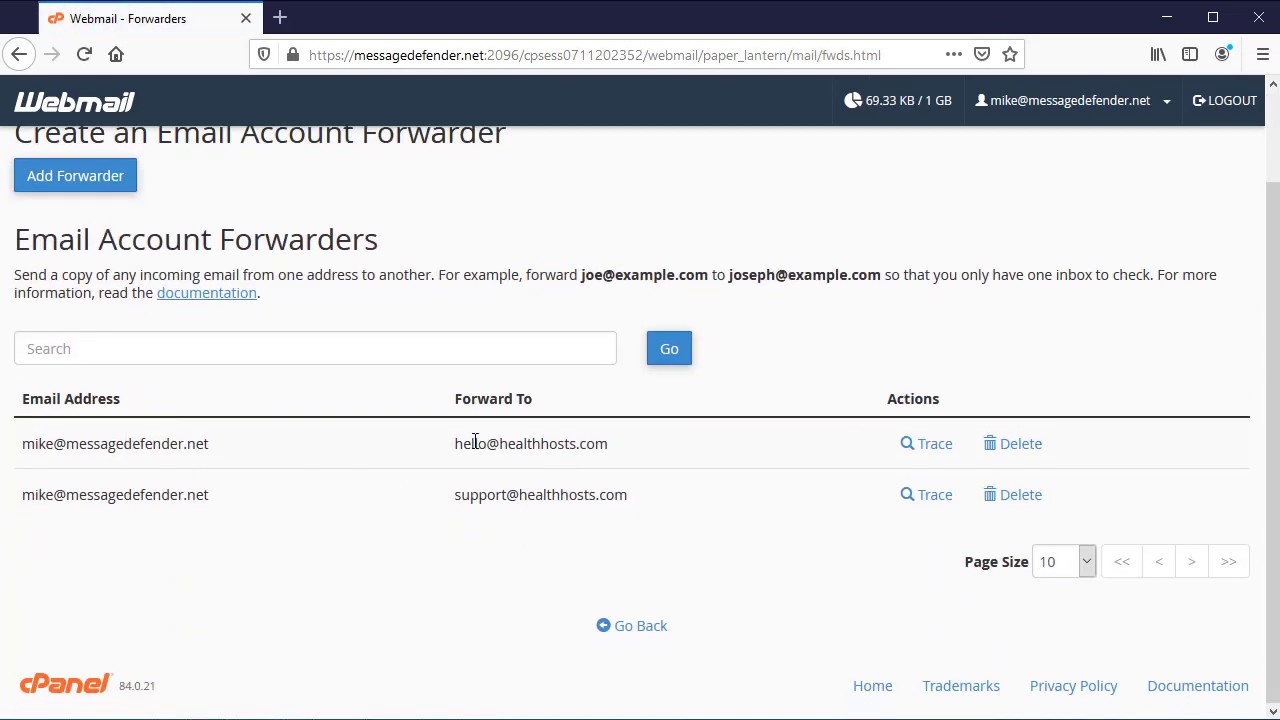This image is a detailed screenshot from a webmail management website interface. The topmost section features a dark blue, nearly black border about an inch thick. Within this border, there's a small white pop-up tab containing an orange infinity sign angled to the right, followed by the text "Webmail-Forders" in black. Adjacent to this is a black 'X', and further to the right within the blue border, there's a white plus sign. On the far right, there are three symbols: an 'X', a square for maximizing the view, and a minus sign for minimizing.

Directly below this is a light gray border with various navigation icons on the left, including a back arrow within a gray circle, a forward arrow, a refresh icon, and a home icon. The central area features a long search bar displaying 'MessageDefender.net', accompanied by an ellipsis, a shield icon, and a star. On the far right of the bar, there are three stacked black lines (a menu icon), a profile icon, a square resembling a book, and four lines ascending with the rightmost line leaning into the others.

A darker gray border follows, split into two parts: on the left, a dark blue section with the text "Webmail" in bold white, and on the right, the text "Logout". Moving leftwards from "Logout", it displays "Mike's email from MessageDefender". Here, there is a circular icon divided in the top right corner with a line extending down and over, indicating storage usage in KBs or GBs.

The main section below is light gray and starts with a large black-printed title: "Create an Email Account Forwarder". Beneath it is a blue button labeled "Add Forwarder" in white. Below, another header in black text reads "Email Account Forwarder", followed by two lines of information fields. Another long search bar is placed underneath, with a centered blue button labeled "Go" in white. Further down, there are columns labeled "Email Address" on the left, "Forward to" in the middle, and "Actions" on the right, with two entries listed below these labels.

At the bottom left corner, there is a small green "cPANEL" logo, while the bottom right section lists several links in blue: "Documentation", "Privacy Policy", "Trademarks", and "Home", all arranged from right to left.